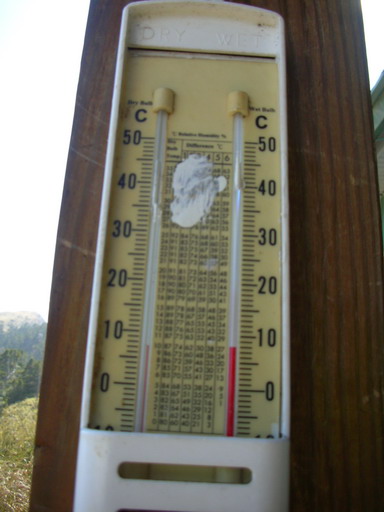This image captures a detailed view of an outdoor thermometer device mounted on a robust, dark-stained wooden post, which could likely be a corner fence post. The device, made of a cream-colored plastic with black inscriptions, features two side-by-side thermometers on a single unit. Each thermometer displays temperatures in Celsius, with both gauges indicating the same reading. Between them, a central panel likely shows a Fahrenheit conversion chart, enhancing the usability of the instrument. The background subtly reveals a scenic landscape, with glimpses of a forest and distant mountains, adding a natural context to the setting.